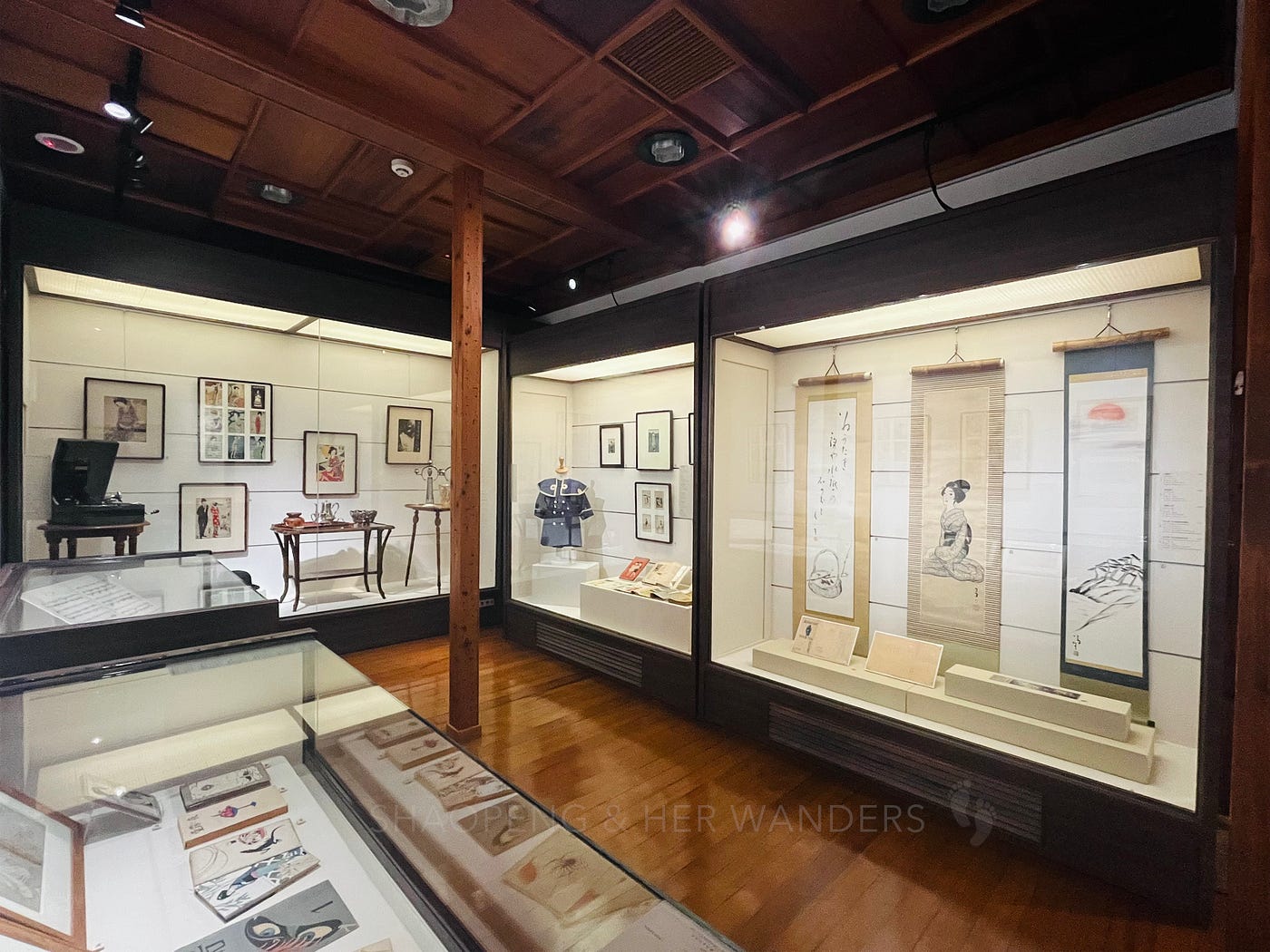This detailed photograph captures the intricate interior of a Japanese-themed art museum. The room features polished medium brown wooden flooring and a matching ceiling, creating a warm, natural ambiance. A slender wooden pillar stretches from floor to ceiling, adding to the architectural elegance. In the background, there's a vintage black record player, and illustrated pictures of Japanese individuals adorn the walls, dressed in various traditional outfits and suits.

Prominently displayed are several glass cases containing an array of exhibits. One glass case, resembling a table, showcases a beautiful tea set and what appears to be a child's outfit from a bygone era. Other cases feature Japanese calligraphy scrolls and framed paintings, meticulously lit to emphasize their artistic details. Long, intricately designed tapestries hang, illustrating traditional Japanese artistry.

In the middle of the room, three Japanese scrolls are unfurled, providing a captivating centerpiece among the other framed artworks. The exhibits are accompanied by detailed descriptions, helping visitors understand the cultural significance of each piece. Across the middle of the image, a logo reads, "Shopping in Her Wonders," hinting at a possibly interactive or themed segment of the museum display.